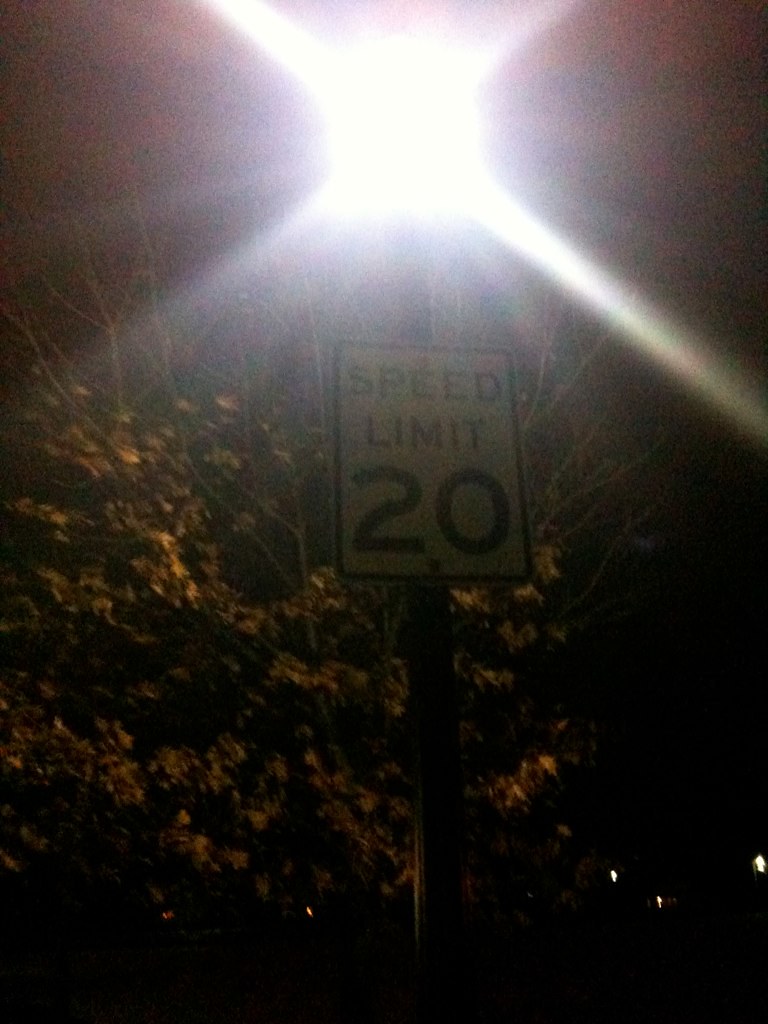This nighttime photograph captures a close-up of a street light illuminated against the dark sky. The bright glow of the street light creates a noticeable glare on the camera lens, emphasizing its intensity. Directly beneath the light, a speed limit sign prominently displays "20" in bold black numbers on a standard white background with a black border. The words "SPEED LIMIT" are written in all capital letters and also in black. Situated behind the sign is a small tree, its branches and sparse foliage tinged with hues of orange, yellow, and hints of green, suggesting a transitional season—either summer waning into fall or spring advancing into summer. The upper branches of the tree are more visible, sparsely covered with leaves, adding an element of natural texture to the scene.